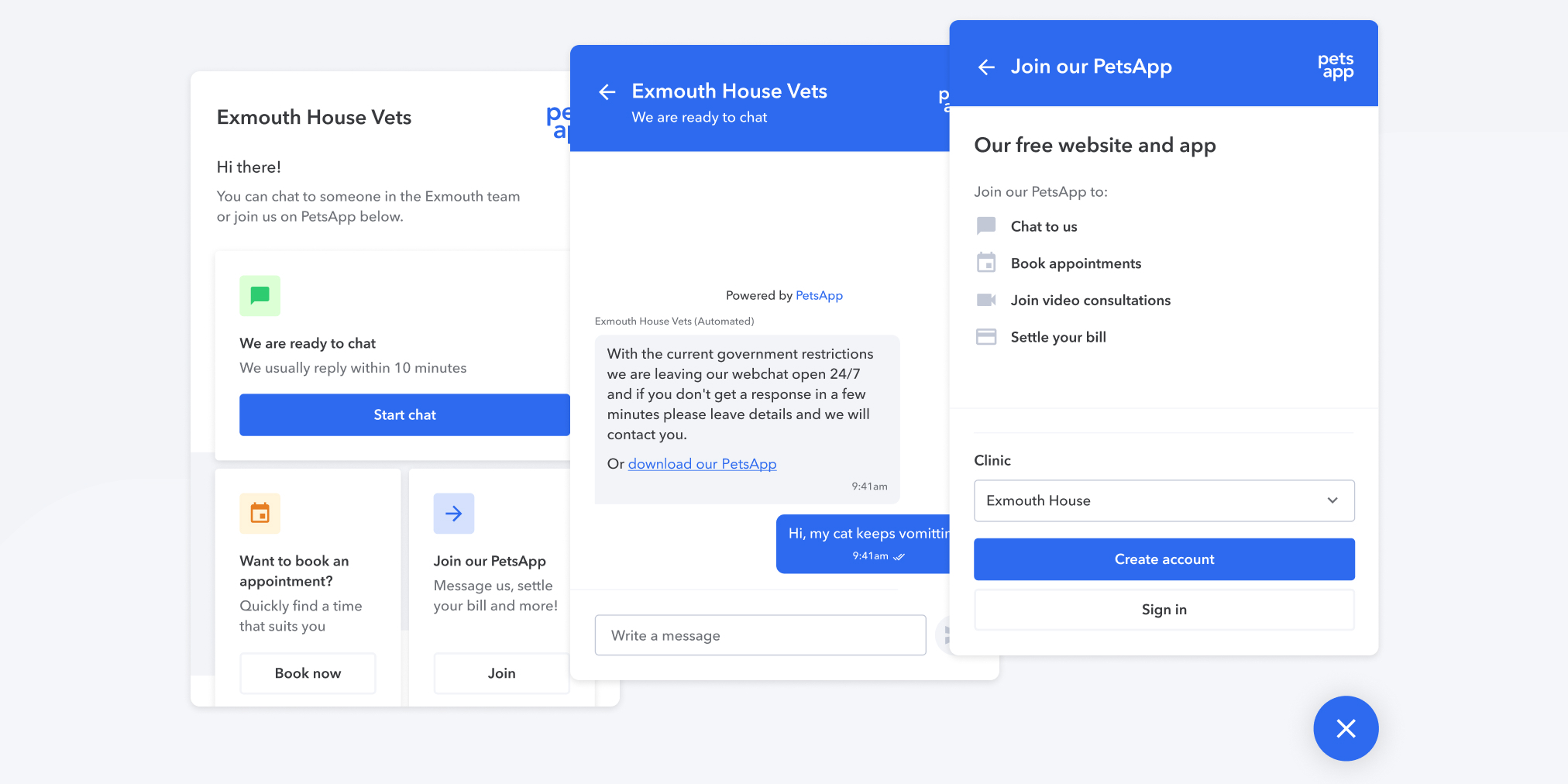Here is a cleaned-up and detailed descriptive caption for the image:

---

The image comprises a stack of three overlapping screenshots from a mobile device, related to xMouth House Vets and their PetSapp service.

**Screenshot 1 (Bottom Layer):**
- **Header:** "xMouth House Vets" displayed prominently.
- **Text:** "Hi there, you can chat to someone in the xMouth team or join us on PetSapp below."
- **Interactive Boxes:**
  1. **Start Chat:** The box spans the entire width of the device, featuring a green cartoon dialogue icon. The button is blue with white text reading "We’re ready to chat, we usually reply within 10 minutes. Start Chat."
  2. **Book an Appointment:** A half-width box with a calendar icon. It says "Quickly find a time that suits you" and has a white button with black text that reads "Book Now."
  3. **Join our PetSapp:** Another half-width box with an arrow icon. It reads "Message us, settle your bill and more," and has a white button with black text reading "Join."
- **Background:** Top 60% in white, bottom 35% in gray, and a small white footer area.
- **Additional Text:** Blue text in the upper right corner, likely reading "PetSapp."

**Screenshot 2 (Middle Layer):**
- **Chat Window:**
  - **Header:** Blue background with white text, showing a back arrow and "xMouthHouseVets" along with an obscured PetSapp logo. It states, "We are ready to chat."
  - **Text Content:** "Powered by PetSapp, xMouthHouseVets (automated). With the current government restrictions, we are leaving our web tab open 24-7. If you don't get a response in a few minutes, please leave details and we will contact you or download our PetSapp." The "download our PetSapp" is a clickable link.
  - **Time Stamp:** 9:41 a.m.
  - **Customer Message:** "Hi, my cat keeps vomiting." This message is marked as read with a double check mark.
  - **Input Field:** At the bottom, a text input area labeled "Write a message" and an arrow icon indicating a send button.

**Screenshot 3 (Top Layer):**
- **Join PetSapp Page:**
  - **Header:** Blue background with white text, including a back arrow and "Join our PetSapp" along with a PetSapp logo.
  - **Text Content:** "Our free website and app. Join our PetSapp to chat to us, book appointments, join video consultations, and settle your bill." Accompanied by respective icons: chat, calendar, video, and credit card.
  - **Drop-Down Menu:** "Clinic" menu option with xMouthHouse selected.
  - **Buttons:** Two buttons at the bottom— a blue button with white text "Create Account" and a white button with black text "Sign In."

The background across the screenshots is gray. Additionally, there is a round blue button with a white 'x' in the lower right corner of the image.

---

This caption provides a clear and detailed description of the three screenshots, ensuring all elements are accurately depicted.